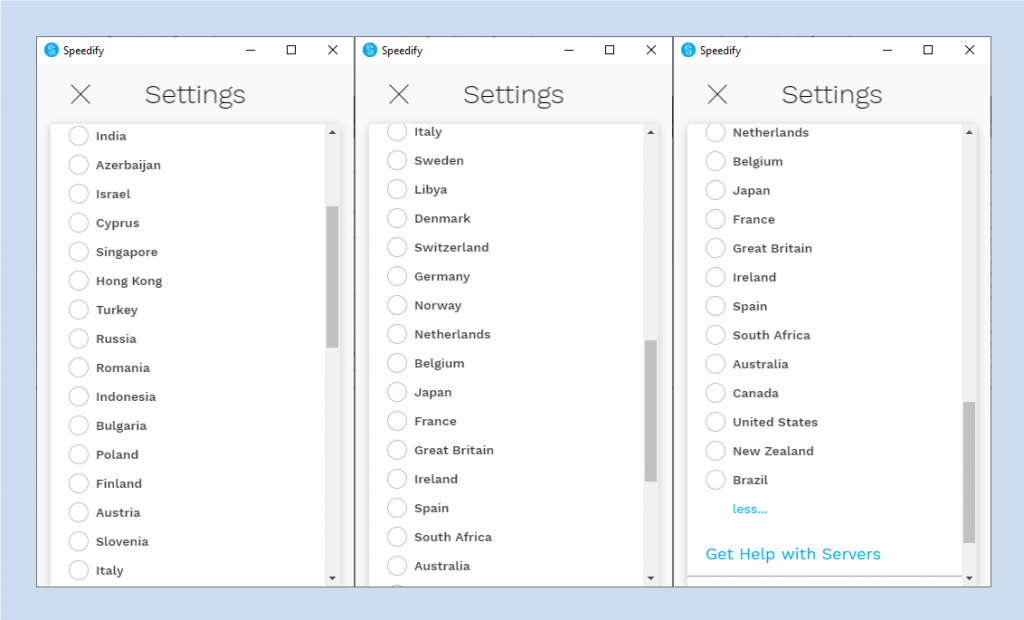A set of screenshots displaying the "Settings" menu for the Speedify application. 

The first screenshot showcases a list of countries starting from top to bottom: India, Azerbaijan, Israel, Cyprus, Singapore, Hong Kong, Turkey, Russia, Romania, Indonesia, Bulgaria, Poland, Finland, Austria, Slovenia, and Italy.

The middle screenshot continues with the countries, starting from Italy, followed by Sweden, Libya, Denmark, Switzerland, Germany, Norway, Netherlands, Belgium, Japan, France, Great Britain, Ireland, Spain, South Africa, and Australia.

The final screenshot repeats "Settings" at the top and lists the following countries: Netherlands, Belgium, Japan, France, Great Britain, Ireland, Spain, South Africa, Australia, Canada, United States, New Zealand, and Brazil. Beneath this list, there is an option labeled "Less..." followed by a prompt to "Get help with servers."